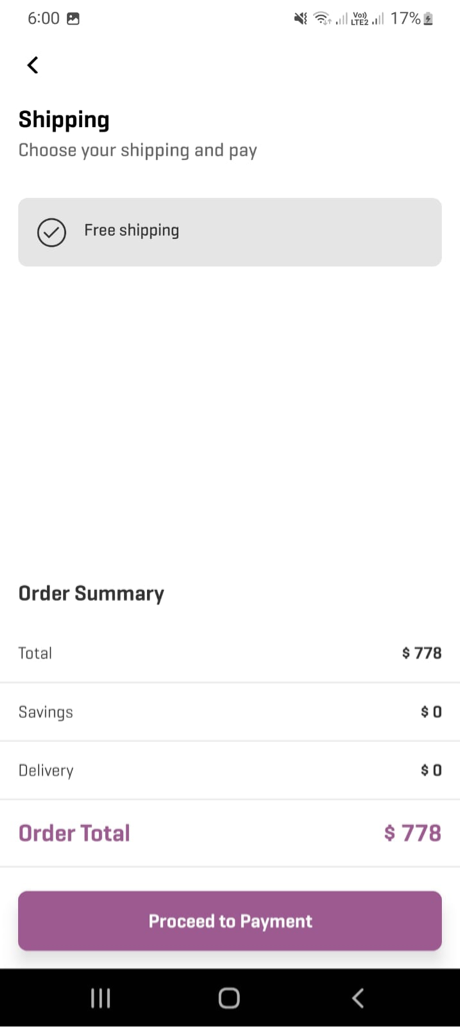In the screenshot captured from a phone, the time displayed in the upper left-hand corner reads 6 o'clock. On the upper right-hand corner, a charging battery symbol shows a 17% charge. Below this, on the left side, the text reads "Shipping. Choose your shipping and pay." Immediately beneath that, a gray pop-up bar indicates "Free Shipping" with a checkmark symbol to its left.

Following this is a section of blank white space, before reaching the "Order Summary" located towards the bottom left of the screen. This section details the following:
- The first line reads "Total" with the corresponding amount "$778" on the right.
- The next line states "Savings" with an amount of "$0."
- The subsequent line mentions "Delivery," also marked as "$0."
- The final line, labeled "Order Total," reiterates the amount of "$778."

Beneath this summary is a prominent purple button with white text that says "Proceed to Payment". At the very bottom of the screen, there is a black navigation bar containing three buttons: a menu button symbolized by three horizontal lines on the far left, a circular home button in the center, and a back button on the far right.